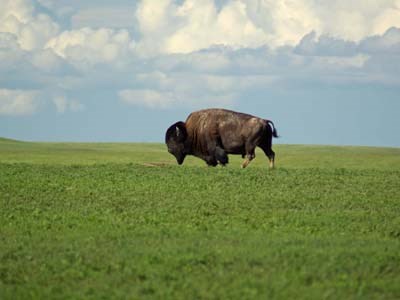The photograph depicts a solitary bison standing in the center of a lush, green meadow, possibly located in the Western United States. The meadow is slightly hilly and covered in vibrant, grassy terrain. The bison, a robust, dark brown creature, features a prominent hump over its shoulders, powerful and muscular build, darker head and beard, and almost black front legs. It appears to be grazing or searching for food amidst the open, tranquil landscape. Above the meadow, the sky is a striking bright blue, scattered with fluffy cumulus clouds interspersed with some storm clouds that reflect sunlight, adding depth and contrast to the scene. The foreground of the image is slightly blurred, emphasizing the bison's placement and the expanse of the meadow. The photograph is professionally taken, capturing the essence of wildlife in its natural habitat.